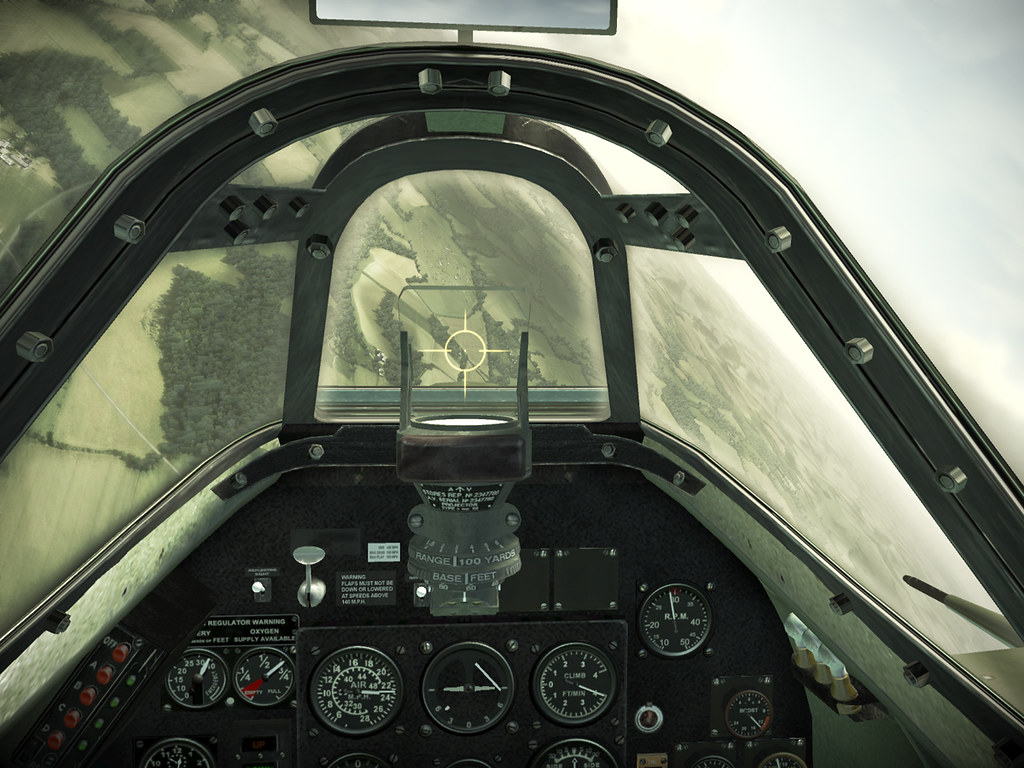The image depicts an immersive view from the cockpit of a World War II-era single-seater fighter jet, likely captured from a highly realistic air combat video game or an advanced AI-generated visualization. The perspective places you directly in the pilot's seat, surrounded by a mechanical interior adorned with multiple circular gauges displaying various flight metrics. These gauges, along with a physically mounted gun sight—featuring a yellow target indicator on a piece of glass—emphasize the hands-on, instrumental nature of piloting the aircraft. The cockpit canopy is constructed from glass panels, connected by metal frames with visible rivets, enveloping the pilot in a protective dome. Outside, the environment is characterized by a subdued, sepia-toned landscape with fields, grass patches, and sparse trees stretching out below, providing a stark contrast to the grayish sky that tilts to the right, indicating the plane is banking left in a descending maneuver. The detailed depiction of the cockpit's instruments and the marked sights on the windshield aligns the pilot's focus on precise targeting amidst the tactical flight.